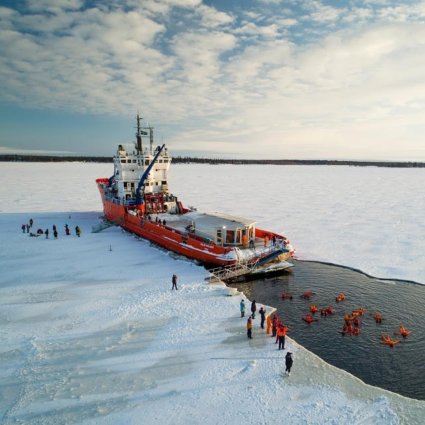This color photograph captures a striking scene in the Arctic or on an icy plain, showcasing a red and white ice-cutter barge with a raised, windowed crew compartment. The vessel has carved a path through the ice, leaving a visible trail of open water that extends from the lower right-hand corner of the image toward the upper left, indicating its movement. The ice field surrounding the ship is vast and barren, with a dark, ambiguous land or tree line barely visible below the cloud line in the distant background. The sky is predominantly cloudy with patches of vibrant blue peeking through, suggesting a clear day without any impending storms. 

On the ice, several groups of people in dark clothing can be seen standing and observing the ship, casting elongated shadows across the frozen surface. Behind the boat, the ice is split, revealing the channel it has forged, where reddish-brown nets or floating debris drift in the water. The ship appears to be momentarily halted, entrapped by the ice that flanks its sides and obstructs its path forward, creating a narrow corridor through which it had been navigating. The overall scene is one of stark, frigid beauty, punctuated by the bold colors and human presence in an expansive, icy wilderness.